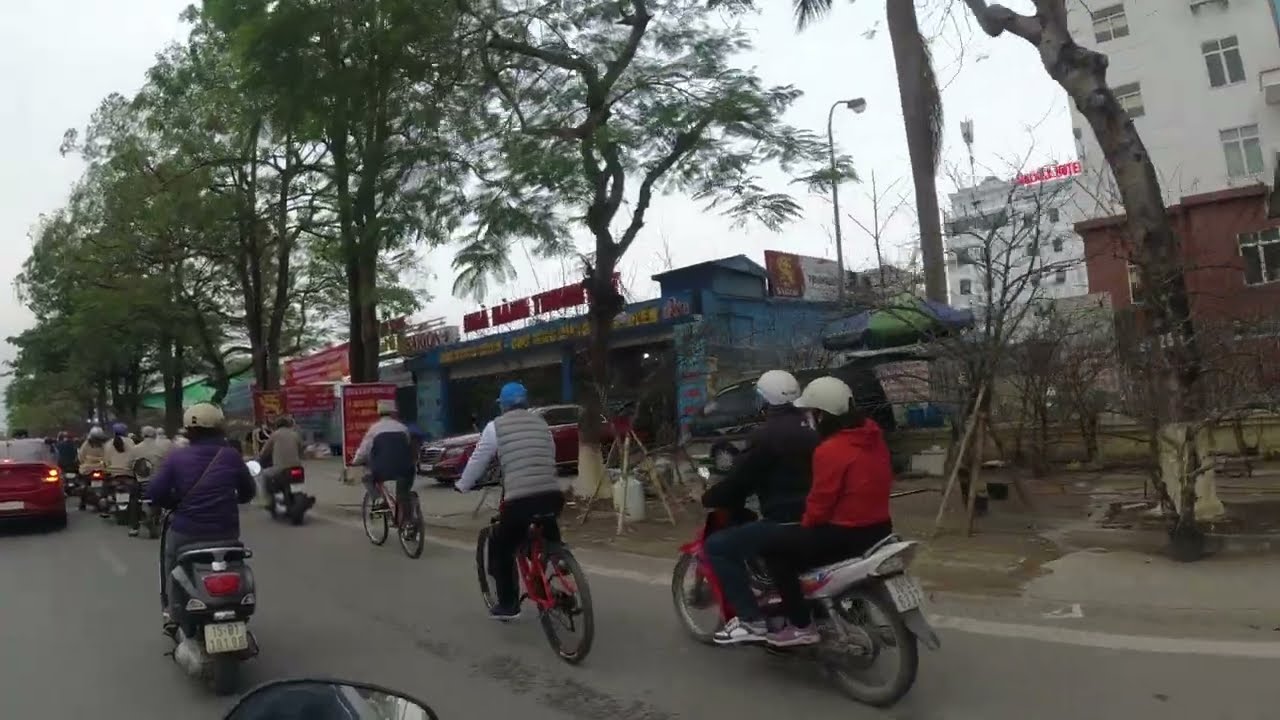The image portrays a bustling Asian street, likely in Vietnam, based on the Vietnamese signage indicating a location possibly in downtown Saigon. The scene is framed by run-down and dirty buildings, with one tall white structure resembling a hotel in the background, accompanied by a shorter red building in front. The street runs westward from the bottom left to the bottom right, lined with seven trees on the left side and a dead tree on the right.

The street is teeming with activity, featuring nine motorcyclists and two bicyclists, all clad in various puffer jackets, including gray and purple. Some riders wear helmets, while others don hats. Prominent among the vehicles is a red car visible to the left, with another red car parked in a driveway next to a blue building with garages and red and yellow signage.

The atmosphere is overcast, suggesting it is mid-day, and while the ground appears clean, the overall ambiance of the photo speaks to a well-worn locality imbued with daily life and movement.